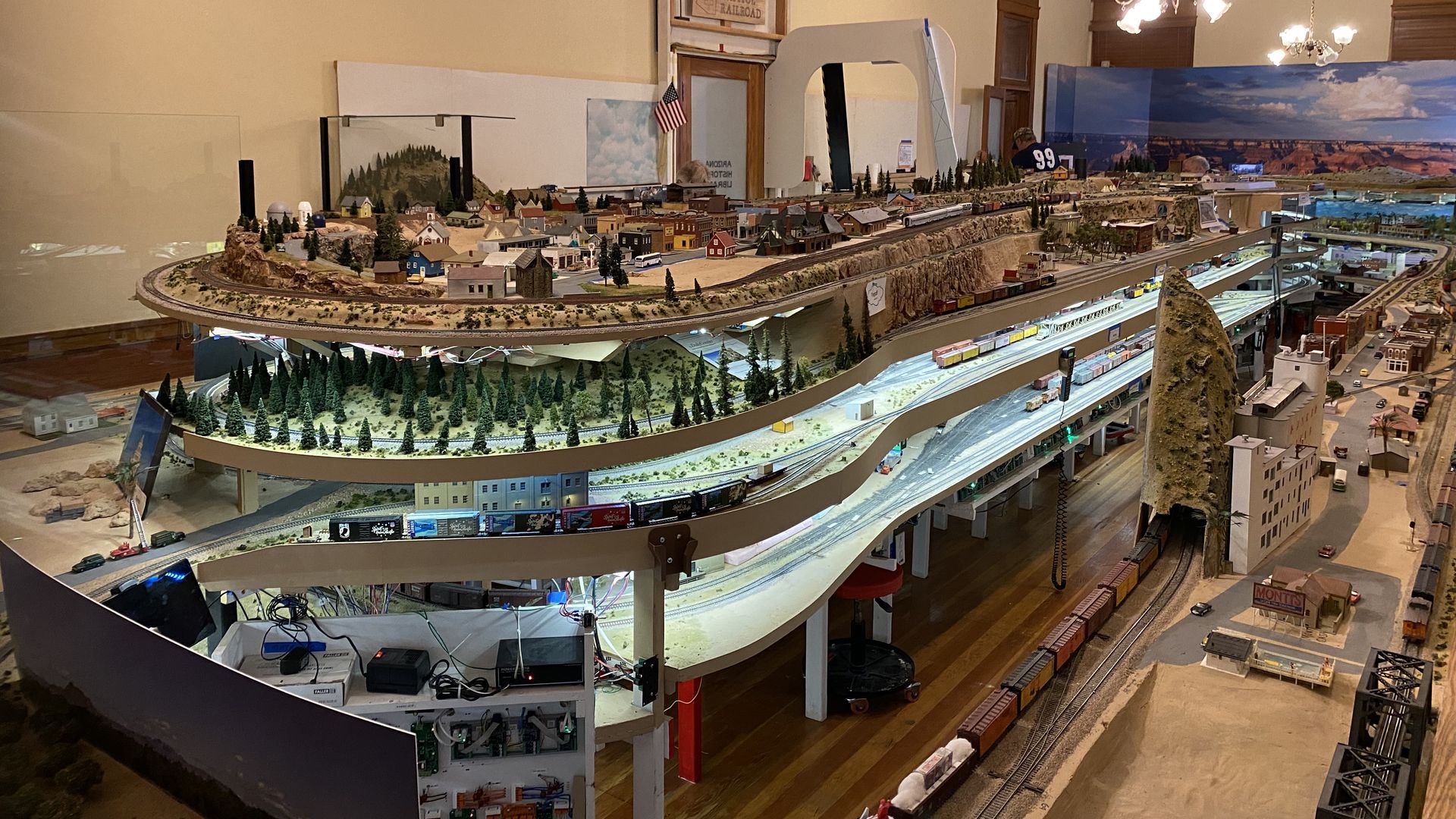This is a horizontally aligned rectangular photograph taken inside a large room, showcasing an intricate and multi-layered model city. The tan-colored wall on the upper left side of the image has a door in the middle with a wooden frame and frosted glass center, adorned with black text. An American flag is hung next to the door, and to its left is artwork depicting clouds. The room's ceiling on the top right corner features lit hanging lights.

In the center of the image dominates a highly detailed five-layered display, portraying a miniature cityscape. The topmost layer presents model houses surrounded by dirt and trees, creating a realistic suburban feel. The second layer is populated with a dense arrangement of trees and a road. Moving down, the third and fourth layers exhibit train tracks complete with model trains in motion, enhancing the dynamic nature of the display. The ground level includes a tunnel, from which a train is emerging, and an array of wires exposed to operate the models. The meticulous recreation includes mini trees, cars, buildings, and flags, encapsulating a comprehensive and impressive depiction of a small town or suburban area.